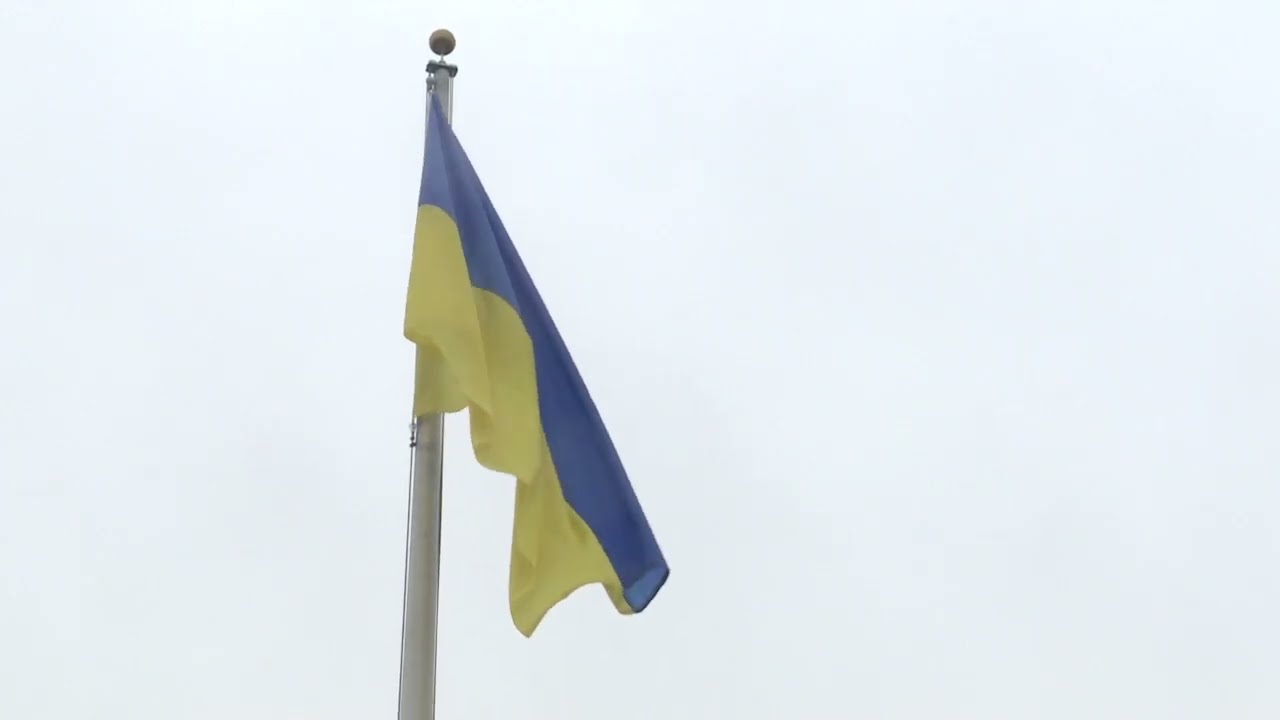This image features a clear, light blue background, suggestive of a bright, cloudless day. Dominating the composition slightly left of center is a vertically extended flagpole, presented in a metallic silver hue. The flagpole is cropped at the bottom, extending close to the frame's apex where it's capped with a dark ball. There are visible strings on the left and right sides of the pole. Suspended from the top of the flagpole is the Ukrainian flag, showcasing its distinctive blue upper half and yellow bottom half. The flag droops limply downward, with a slight tilt, suggesting a lack of wind.